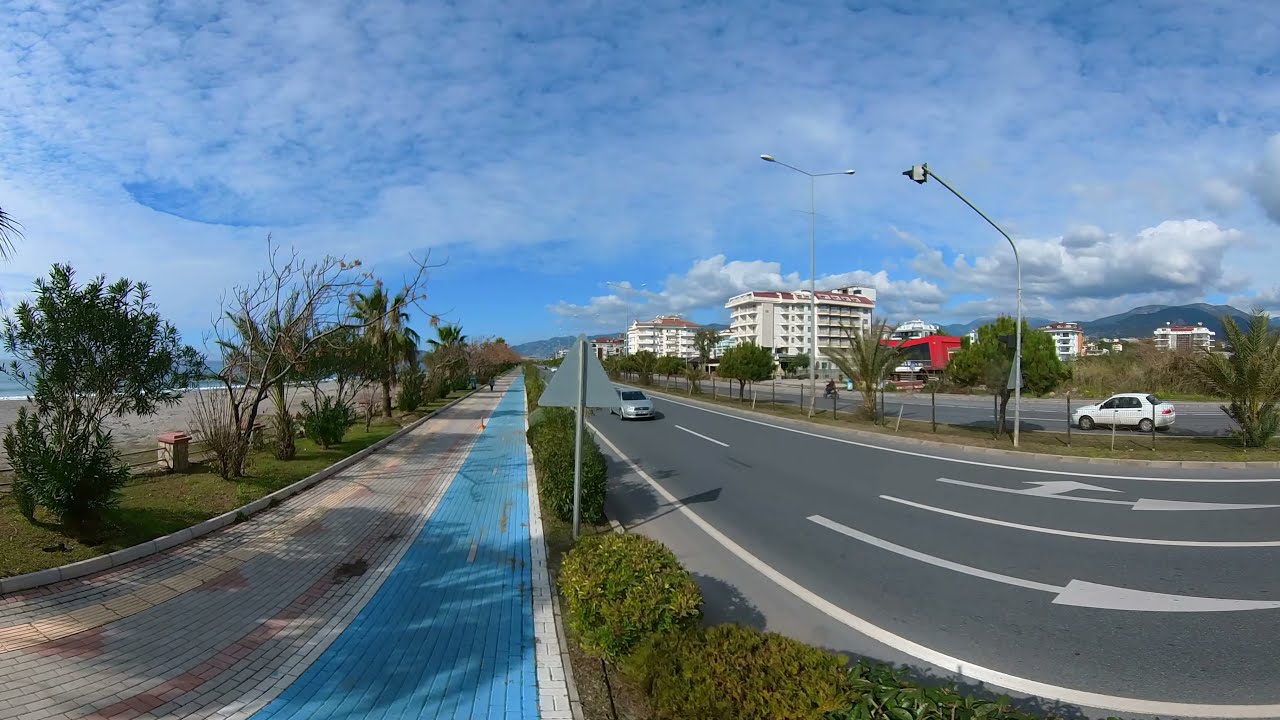The high-angle image, taken from about the same height as a street sign, showcases a scenic coastal area with a distinct fisheye lens distortion. Dominating the scene is a brick-inlaid bike path and footpath that run parallel to a four-lane highway, bordered by a grassy median lined with trees. The bike path, which leads off into the distance, features segregated sections with regular and blue bricks, possibly distinguishing areas for pedestrians and cyclists. On the left, the path is flanked by a strip of grass and trees, leading to a picturesque beach where ocean waves are visible in the distance.

Above, the sky is a serene blue with feathery white clouds, enhancing the idyllic coastal atmosphere. On the right side, the traffic flows in both directions, with a white car heading one way and a silver car the opposite. The highway is marked with clear white dashed and solid lines, alongside directional arrows indicating the flow of traffic. 

In the backdrop, several white buildings with brown roofs, resembling apartments or hotels, are interspersed with red and other white structures. Further enhancing the setting is a majestic mountain range with a blue hue, providing a striking contrast to the scene's predominantly green and blue palette. Overall, the image imparts a quintessential California vibe, emphasizing a well-maintained, exclusive area that balances serene natural beauty with meticulous urban planning.